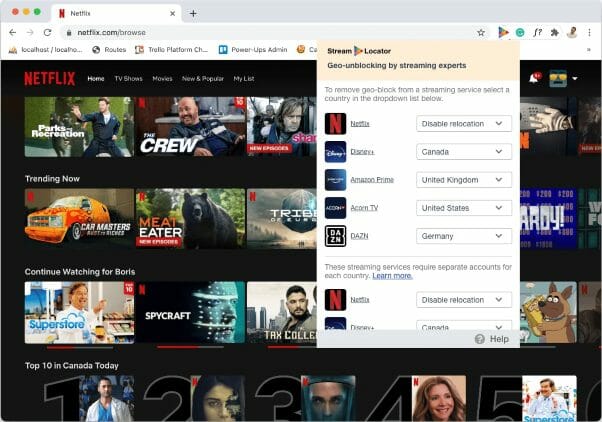The image depicts a screenshot of a web browser on a Mac, displaying the Netflix.com browse page. The browser's bookmark toolbar is densely populated with various saved links, including local host options, routes, Trello, Trello platform, Power-Up admin, and other miscellaneous entries. 

The Netflix interface features its recognizable layout with the red Netflix logo prominently displayed in the top left corner. Navigation options such as Home, TV Shows, Movies, New & Popular, and My List are clearly visible. The content is arranged in multiple horizontal rows, each containing approximately six thumbnails of shows or movies. 

Among the visible thumbnails, popular titles such as "Parks and Recreation," "The Crew," and a documentary called "Man Eater" featuring a bear can be observed. Each thumbnail is accompanied by a photographic representation and the title of the content. 

Below the first row of thumbnails, there is a section labeled "Trending Now," displaying currently popular content. Following this, another row is titled "Continue Watching for Boris," indicating personalized recommendations for the user. Further down, a row named "Top 10 in Canada Today" showcases the most popular shows in the region, ranked from one to ten with corresponding thumbnails.

On the right side of the screen, the thumbnails extend beyond the visible area, suggesting that more content is available by scrolling horizontally. 

Additionally, a large drop-down menu is open on the screen, listing various streaming services such as Netflix, Disney+, Amazon Prime, and Acorn TV. This menu also includes options for different countries like Canada, the United Kingdom, the United States, and Germany. It appears to be part of a geo-unblocking service, with instructions indicating that selecting a country will remove geographic restrictions from a streaming service. The text within the drop-down menu hints that this service may be related to VPN usage, possibly labeled "Geo Unblocking by Streaming Experts."